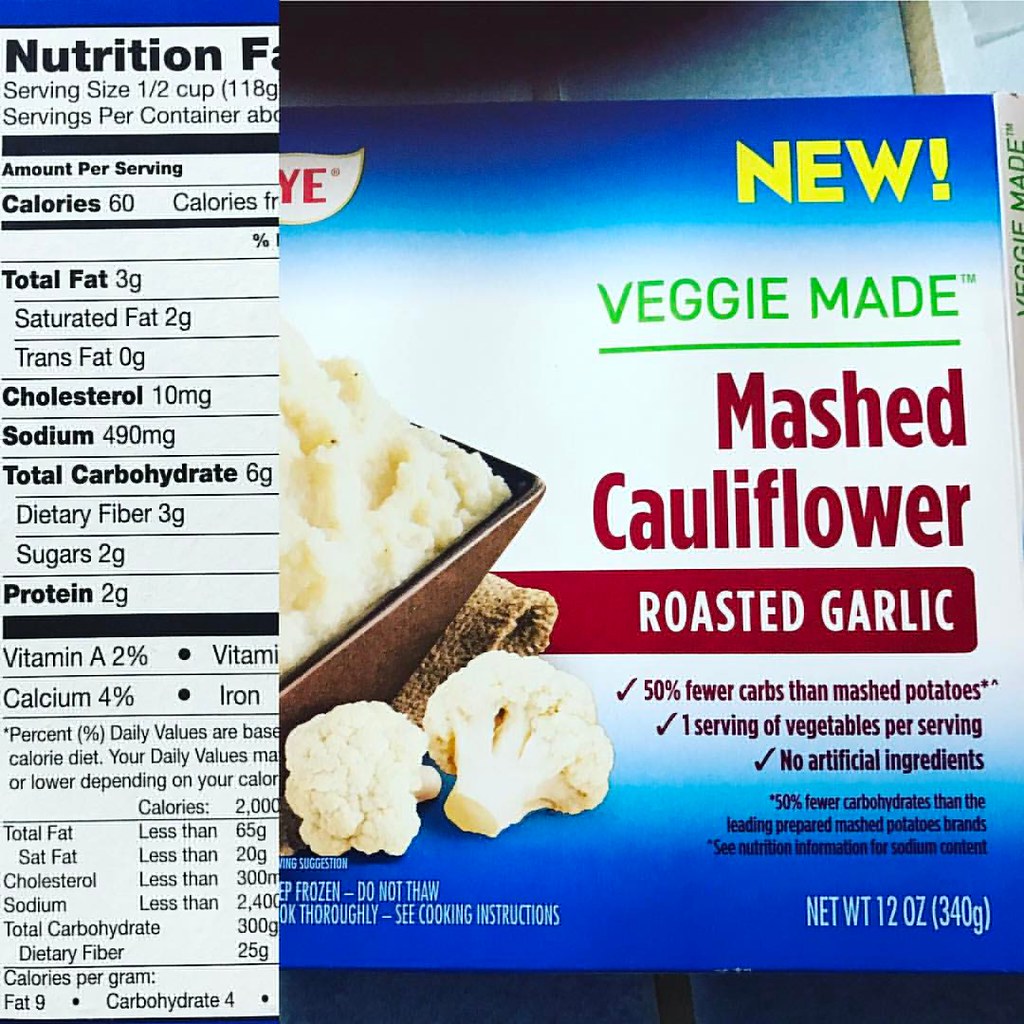A package labeled "Bird's Eye Veggie Made Mashed Cauliflower, Roasted Garlic" is prominently displayed, designed for placement in the vegetable freezer section of a supermarket. The front of the bag features an appealing image of the mashed cauliflower alongside a detailed description highlighting its benefits. The package states it contains 50% fewer carbs than traditional mashed potatoes, provides one serving of vegetables per serving, and contains no artificial ingredients. Detailed nutritional information, including servings per container, vitamins, cholesterol, sodium, and protein content, is visible on the left side of the package. This product offers a healthier, lower-carb alternative to mashed potatoes.